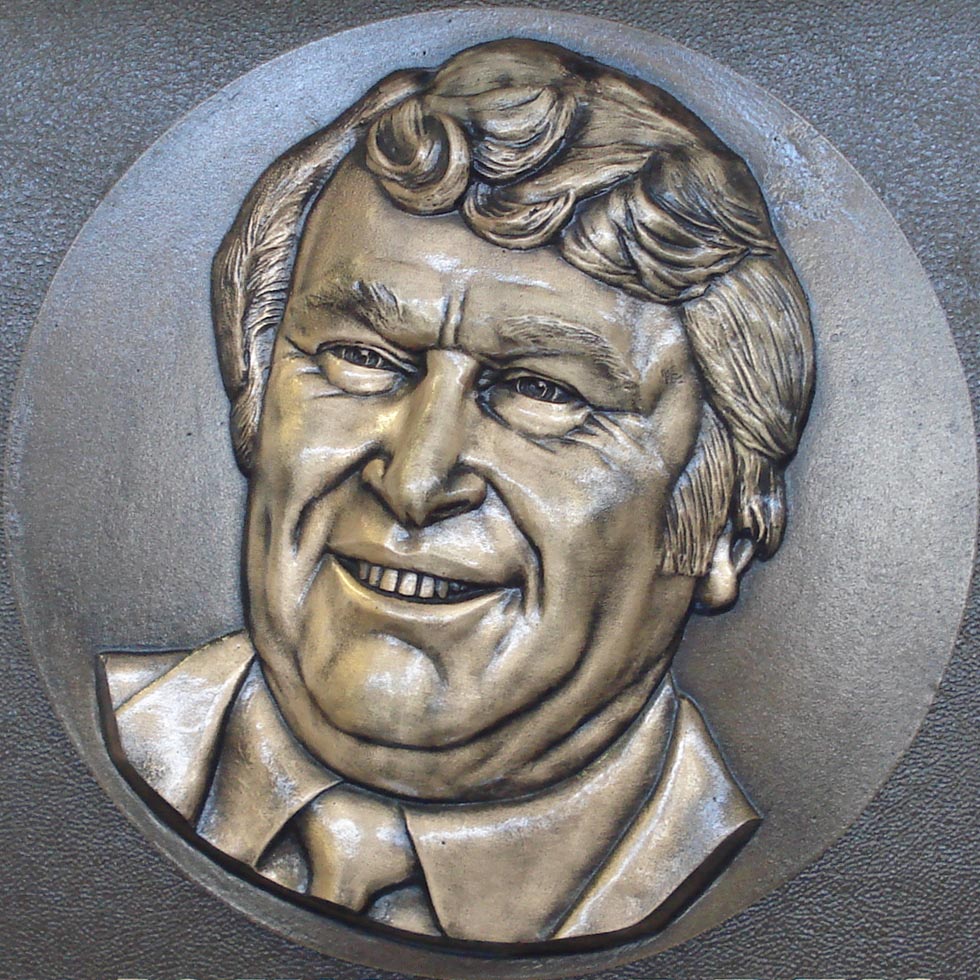This image features a zoomed-in view of a detailed bronze plaque, seemingly positioned outdoors at a monument on a sunny day. The focus is a circular metallic relief prominently placed at the center, depicting the face of an elderly man. The background reveals a textured, likely plaster, brown-and-gray surface that sets off the gleaming bronze. The striking relief showcases the man's distinct facial features: prominent wrinkles around expressive eyes, thick and bushy eyebrows, a long nose, and a wide smile revealing his front teeth. His hair is styled in a 70s fashion—curly on top and straighter on the sides, and he appears to be dressed in a collared shirt, cut off near the neck, suggesting formal attire. Despite the high level of detail, no text is present to identify the individual, leaving his identity unknown, yet suggesting that the intention of this artistic tribute is to honor and immortalize him.